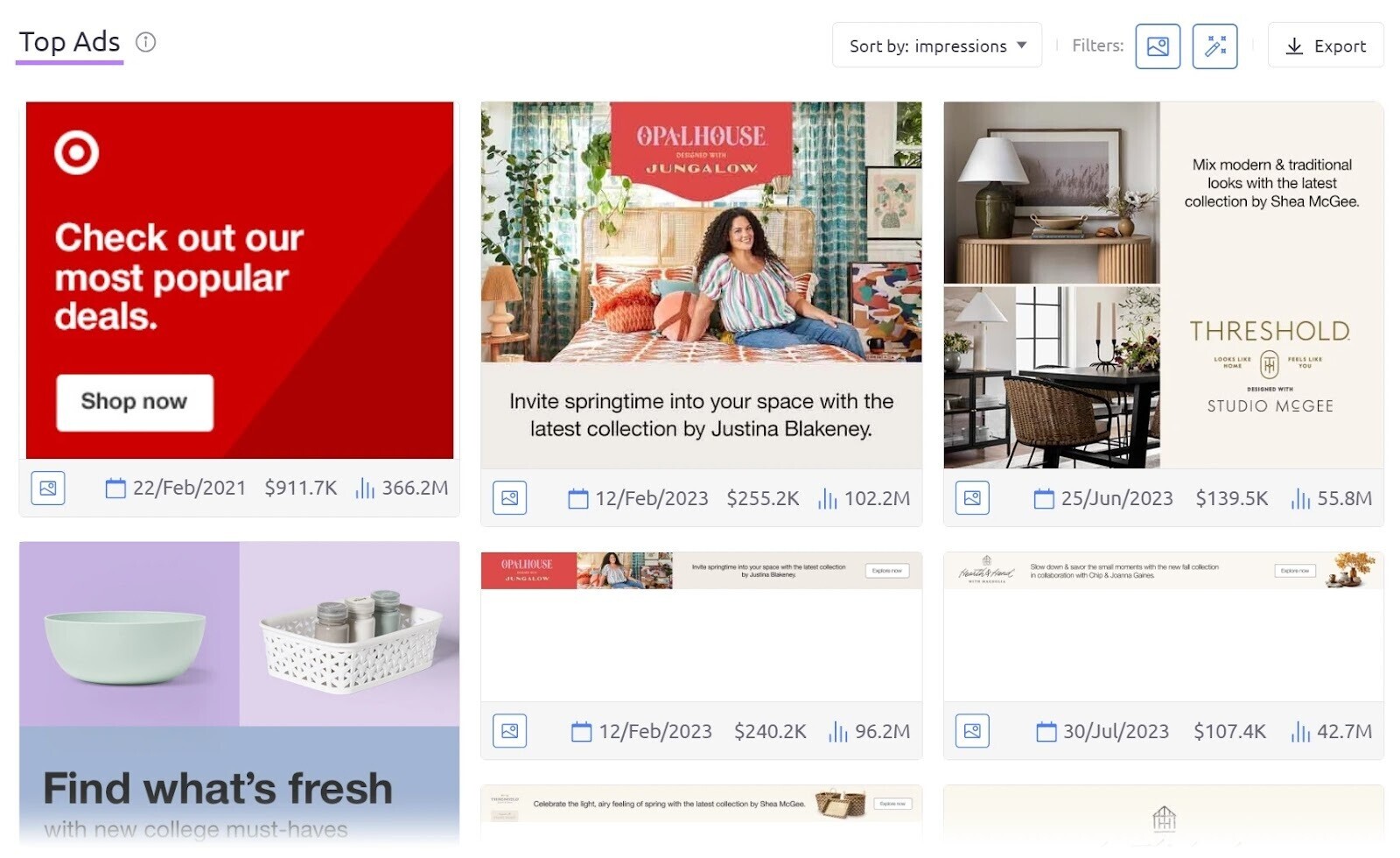The image features a white background with a section titled "Top Ads" in the top left corner, underlined by a thin purple line. To the right of "Top Ads," there's a circle with an exclamation point inside. In the top right corner, a drop-down menu labeled "Sort by: Impressions" is present, adjacent to the gray word "Filters," an icon resembling a sun and mountain, a square icon with a pencil and three stars, and a rectangular button with a downward-facing arrow and "Export" in black.

Below, different ads are displayed. On the left, a red square ad has a white bullseye icon in the top left. Below, it reads "Check out our most popular deals" in white, followed by a "Shop Now" button. Dates, financial figures, and a bar graph icon are also displayed.

Next to it, an ad features a woman with curly brown hair on a bed with blue curtains, bordered by a purplish-red rectangular header reading "Opal House" and "Jungalo" in white. A gray-tan rectangle at the bottom says, "Invite Springtime into your space with the latest collection by Justina Blakeney." Below, date, dollar amount, and line graph data are listed.

To the right, a square ad shows a lamp and a dining table on the left, accompanied by a tan box with black text stating, "Mix Modern and Traditional Looks with the latest collection by Shea McGee," followed by "Threshold" and "Studio McGee" in dark black-brown text. Below, a light gray box lists date, dollar amount, and line chart info.

Further down, another ad row shows colorful boxes: purple, pink, lavender, and a blue rectangle with a bowl, basket with shakers, and "Find What's Fresh with New College Must-Haves" text.

Smaller banner ads are also visible. One features a red rectangle and a dark-haired woman on a bed, with a gray box below showing date, dollar amount, and line graph data. Another banner with a tan background has cursive text, small black text in the center, and a button with black text. Below, a gray box displays date, financial figures, and line graph info.